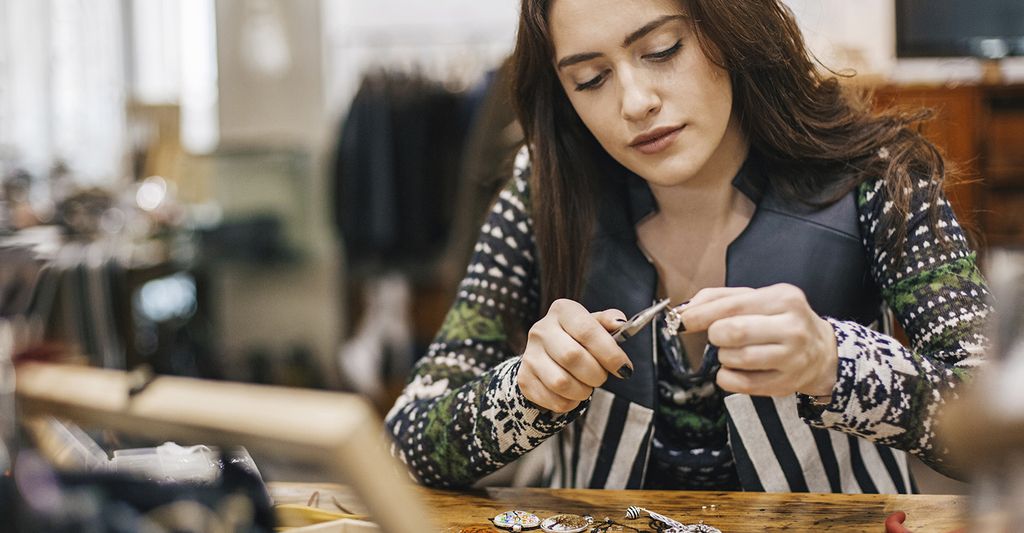The indoor photo captures a woman in her late 20s or early 30s, sitting at a wooden table, deeply focused on crafting a piece of jewelry. She holds a narrow needle or wire between her thumb and index finger, while her other hand skillfully maneuvers a pair of needle-nose pliers. She has long brunette hair flowing beyond her shoulders, her nails painted black, and she wears light makeup with a hint of lipstick. Dressed in a unique ensemble featuring a vest with blue and white stripes and a black top, complemented by a sweater with intricate, colorful patterns of green, dark tones, and possibly snowflakes and stars, she emanates a fun, alternative style. Various beads, wires, and jewelry-making tools are scattered on the table before her, highlighting her meticulous craftwork. The blurred background suggests a classroom or college setting illuminated by natural light streaming through windows, with a TV faintly visible, ensuring the focus remains on her and her intricate work.